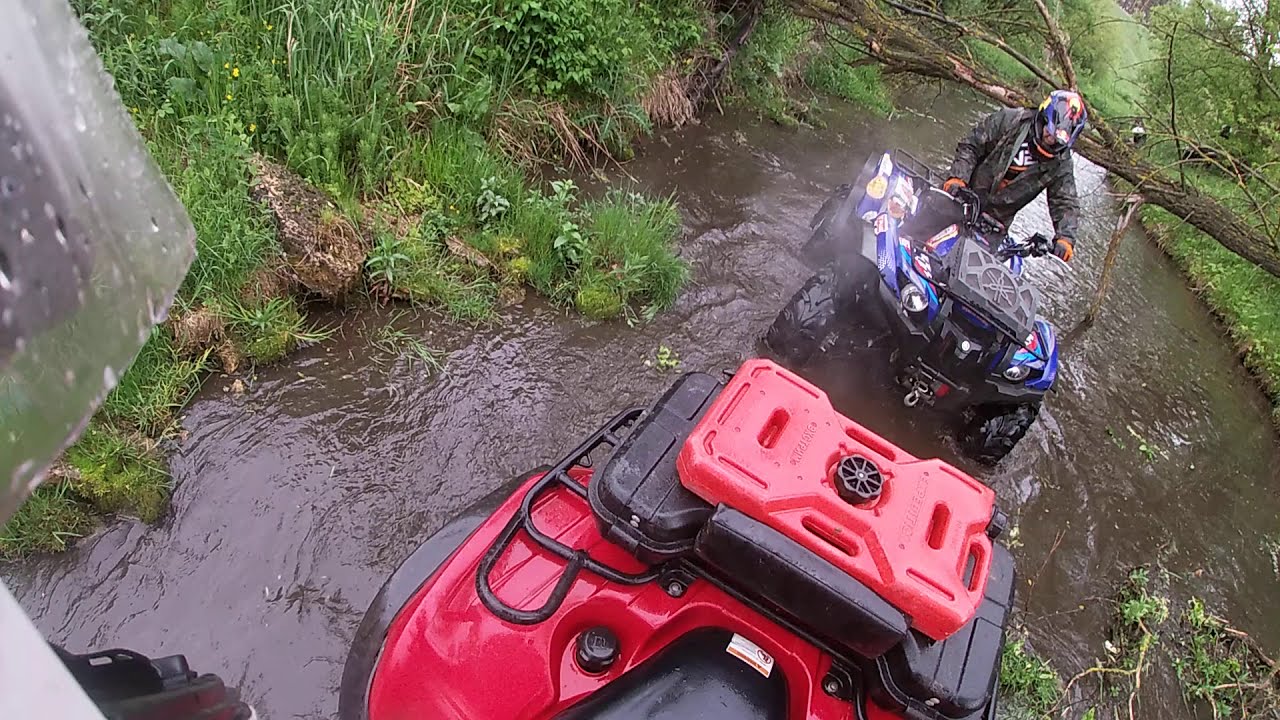In this detailed image, a winding, shallow river is nestled within a lush, verdant landscape brimming with green vegetation. On either side of the river, thick grasses, overgrown leaves, and native plants create a dense forest backdrop. Prominently, a fallen tree stretches across the right section of the river, adding an element of wildness to the scene.

Two ATVs are navigating the shallow, murky, brown waters of the river. The wheels of the vehicles are partially submerged, with water reaching only about a quarter of the way up. In the foreground, a blue ATV with large black wheels is driven by a man clad in a dark camo jacket, orange gloves, and a blue helmet, standing as he grips the handlebars. The blue ATV follows closely behind a red ATV, of which only the rear half, including the gas tank and luggage rack, is visible. The presence of a helmet's glass to the left suggests another rider possibly looking back.

The vivid colors in the image - green foliage, the blue and red of the ATVs, and touches of orange, yellow, and brown - stand out distinctly, painting a scene of adventure and exploration deep within the wilderness.